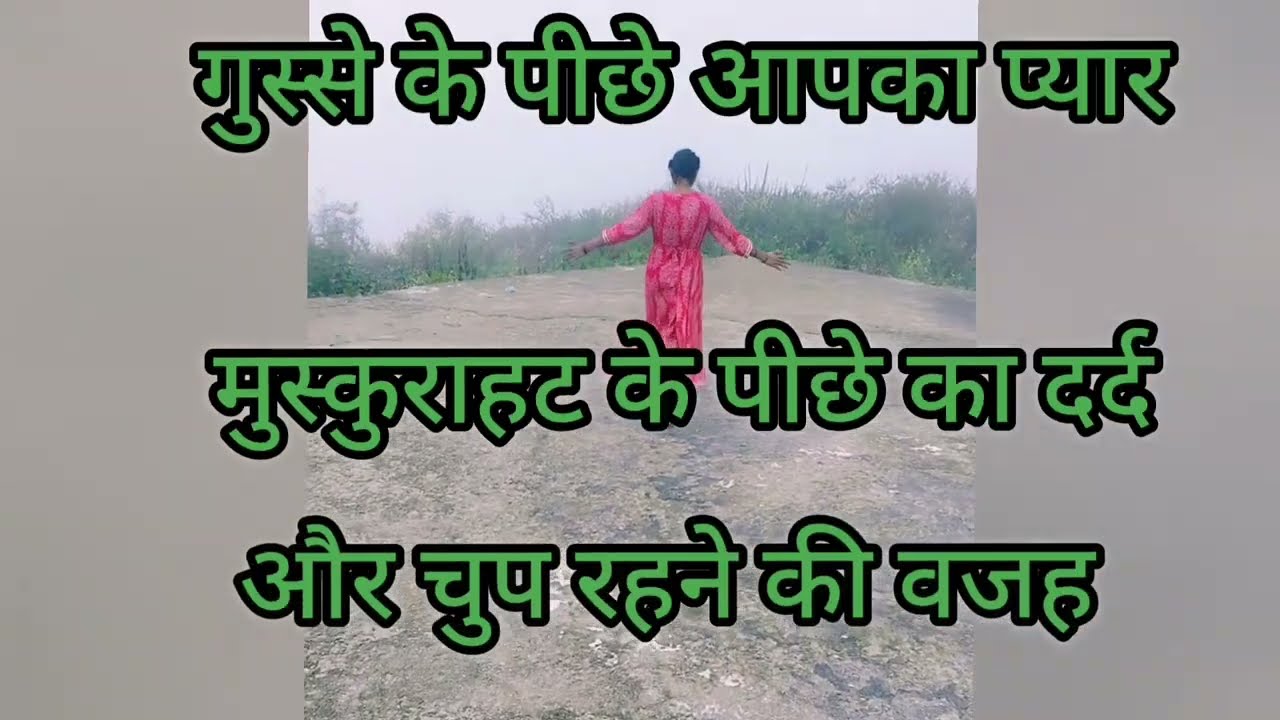The image captures an Indian woman walking down a stone road with lush greenery comprising bushes and tall grass on either side. The sky above is a cloudy, white expanse, setting a serene backdrop. The woman, with dark brown skin and black hair, is donning an elegant red and white dress that reaches her feet. Her arms are outstretched to her sides, and her back is turned towards the camera. Overlaying the image are three rows of green text with a black border, written in a non-English language, likely from the Indian subcontinent. The central image is framed with grey borders on both sides, creating a square format. The scene is a harmonious blend of natural elements and cultural aesthetics.